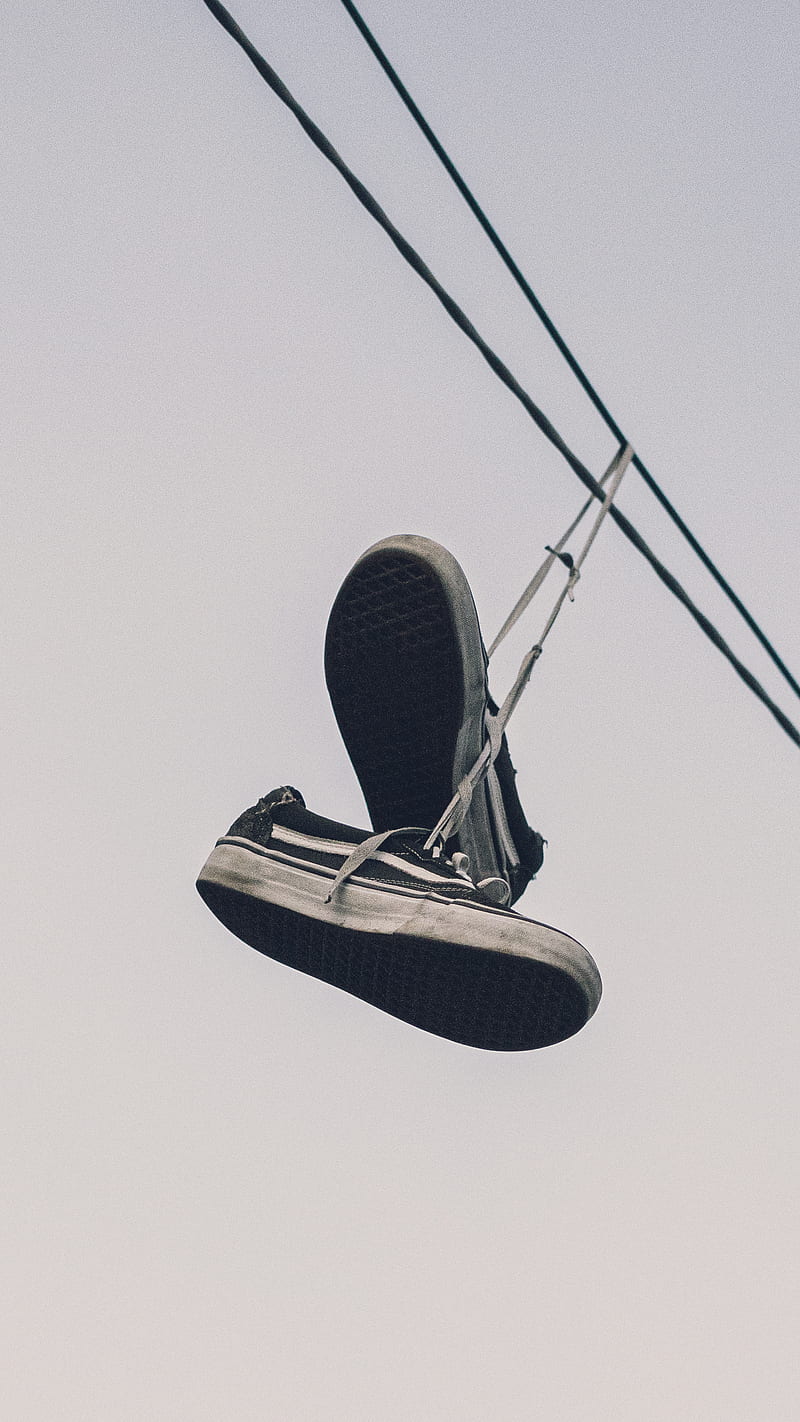The image features an old, black and white pair of canvas sneakers with thick rubber soles, tied together by their shoelaces and hanging from a thin telephone wire or power line. One shoe faces one direction while the other faces another, creating a dynamic composition. The background is a cloudless or fully overcast gray-white sky, giving the impression of an early morning or late evening with no other objects or text visible. This close-up shot captures the worn sneakers with white bottoms and a distinctive white stripe along the sides, suspended against the simple, muted backdrop of the sky.